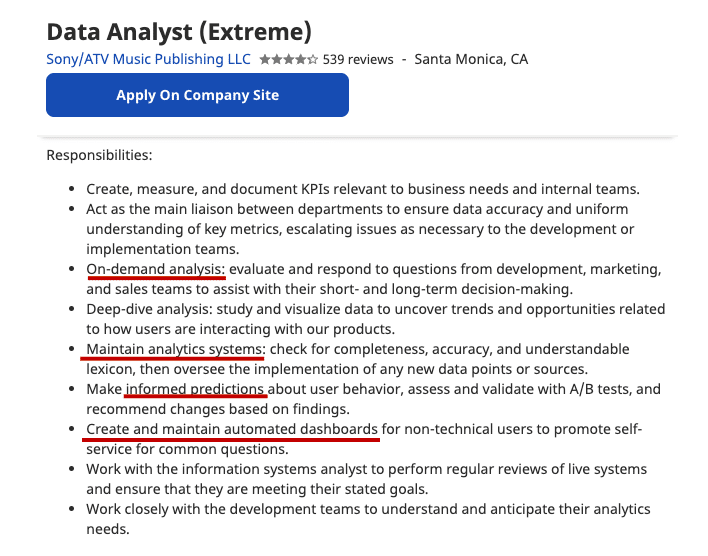**Job Position: Analyst Extreme at Sunny, ATV Music Publishing**

**Location:** Santa Monica, California

**Job Description:**

We are looking for an Analyst Extreme to join our team at Sunny, ATV Music Publishing in Santa Monica, California. This role involves a wide range of responsibilities to support the company’s internal and external data needs. The ideal candidate will:

- **Create, Measure, and Document KPIs:** Develop and monitor key performance indicators that align with various business needs and internal team functions.
- **Liaison Between Departments:** Act as the central point of contact between departments to ensure data accuracy and a uniform understanding of metrics. Escalate issues to relevant development teams when necessary.
- **On-Demand Analysis:** Provide analytical support to the development, marketing, and sales teams. Assist with short-term and long-term decision-making processes by responding to their analytical queries.
- **Deep Dive Analysis:** Perform in-depth studies to visualize data, uncover trends, and identify opportunities through user interaction with products. Ensure these analyses are comprehensible and actionable.
- **Maintain Analytics Systems:** Regularly check the completeness and accuracy of analytics systems. Oversee the implementation of new data sources and maintain a clear, understandable lexicon for data terms.
- **Informed Predictions:** Make informed predictions about user behaviors and validate them with A/B tests. Recommend changes based on findings to optimize future user interactions.
- **Automated Dashboards:** Create and maintain automated dashboards to enable self-service data inquiries for non-technical users. These dashboards should promote easy access to vital information.
- **System Reviews:** Work closely with development teams to understand and anticipate their analytical needs. Perform regular reviews of live systems to ensure they meet their stated goals.

**Applications:** Interested candidates are encouraged to apply via the company’s website.

With over 539 reviews, STARS provides insight into the company culture and employee satisfaction at Sunny, ATV Music Publishing—an exceptional place to nurture a career in data analysis.